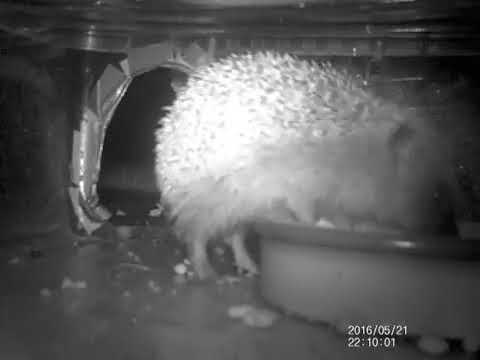In this black-and-white still from a security camera, dated 2016/05/21 at 22:10:01, we see a hedgehog captured in a candid moment. The hedgehog, positioned right of center, dominates the right side of the image with a side profile. Its front legs and nose are deep inside a small bowl, indicating that it is in the midst of eating, while its back legs remain on the ground. The front half of its body is raised, likely due to its spiked back. 

To the left of the hedgehog, there is a small archway or doorway, which appears to be makeshift, possibly taped into place, suggesting a DIY environment made for the hedgehog. The ground around the creature is littered with bits of debris and food. The timestamp on the bottom right corner of the image, appearing in white font, confirms the scene's date and time, adding a poignant touch to this nocturnal snapshot. There's a noticeable light source from the left, illuminating the hedgehog's back and emphasizing the improvised nature of its nighttime habitat.